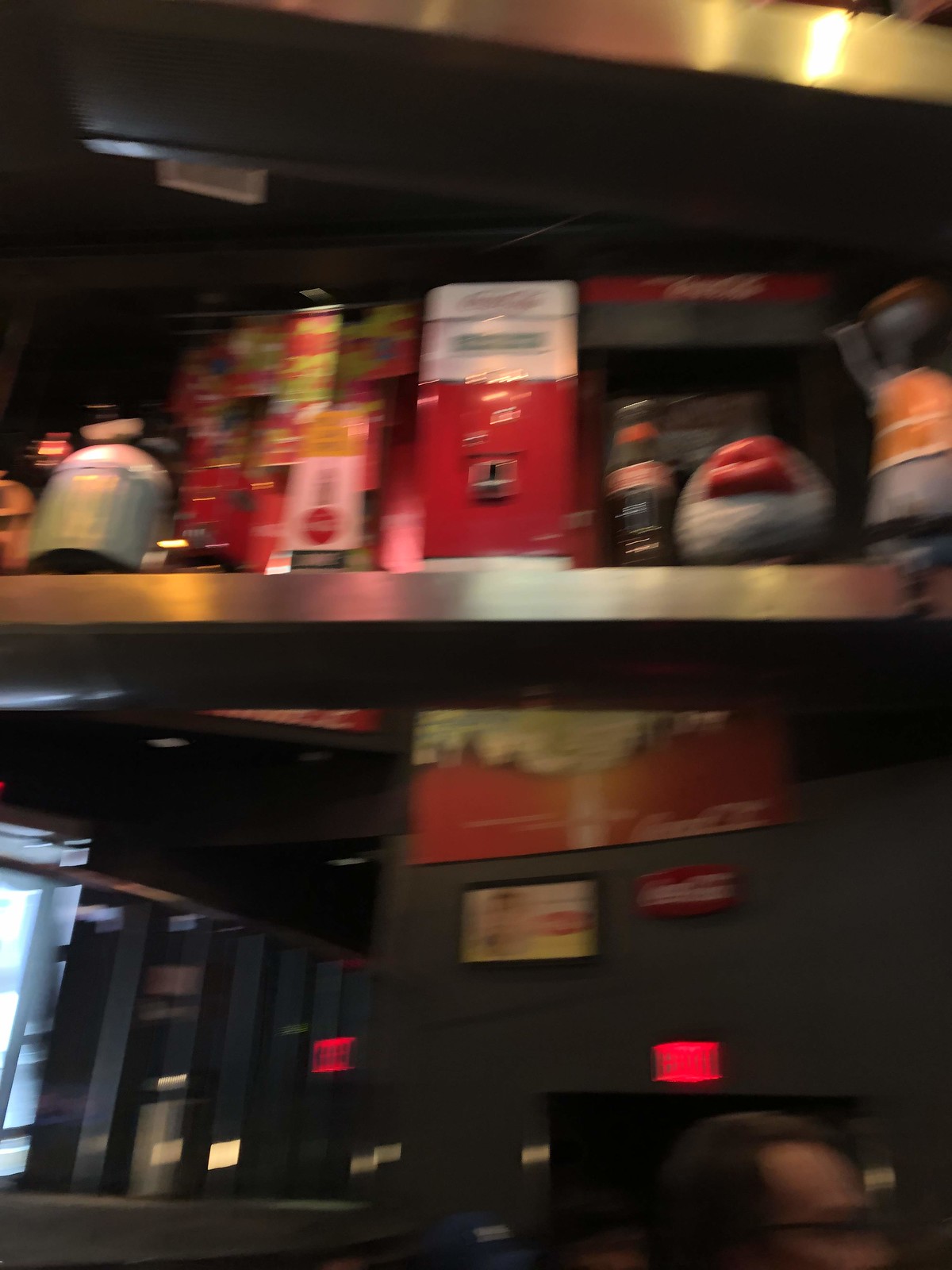This indoor photograph, though slightly out of focus, appears to have been taken in a restaurant adorned with various food-related decorations. The shot is from an unusual angle, capturing the tops of people's heads. Prominently featured is a man with brown hair and glasses, who appears to be Caucasian. Behind him, a person wearing a blue ball cap is partially visible. To the right of them, an exit sign is mounted above a door set against a gray wall.

Highlighting the restaurant theme, the walls are decorated with a vintage red and white Coca-Cola sign, as well as a Lipton tea advertisement. Above the man’s head, a shelf bearing a range of food products and advertisements is visible, albeit slightly blurry. Among the assorted items on the shelf, a silver canister stands out. The decor and ambiance collectively evoke a nostalgic, diner-like atmosphere, indicating the establishment’s focus on food and beverages.